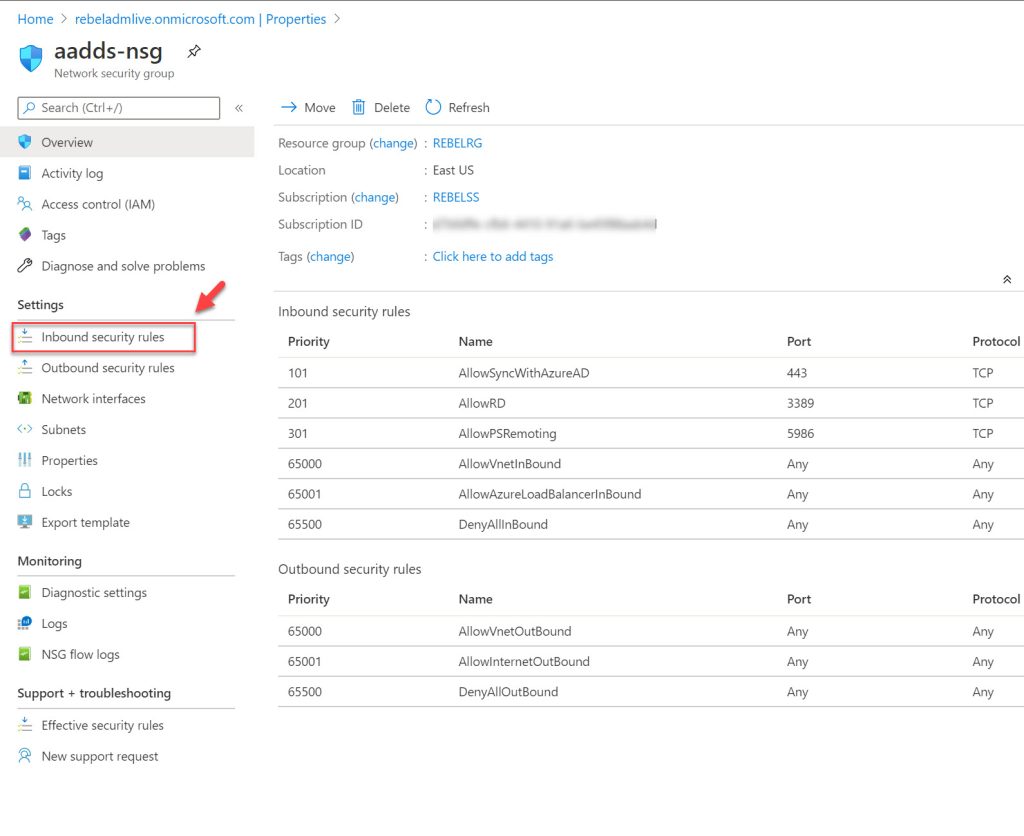The image captures the properties of a Network Security Group (NSG) for a Microsoft account, specifically under the domain rebeladminlive.onmicrosoft.com. The top left corner shows a breadcrumb navigation with a "Home" icon leading to rebeladminlive.onmicrosoft.com. A solid bar separates this from the "Properties" tab, indicating the current view.

On the left panel, a variety of options are presented, including "Overview," "Activity Log," and "Diagnose and Solve Problems," among others. The current view appears to be under the "Settings" tab, particularly focusing on "Inbound Security Rules."

The main section of the image displays detailed information about the security rules. At the top, key properties include:
- **Resource Group**: rebelrg
- **Location**: East US
- **Subscription**: rebelss
- **Subscription ID**: (blurred)
- **Tags**: None listed

For both "Inbound Security Rules" and "Outbound Security Rules," the rules are organized into columns:
- **Priority**: Numerical values indicating the order of rule application.
- **Name**: Names assigned to each rule.
- **Port**: Ranges from specific numbers to the term "Any."
- **Protocol**: Specifies either "TCP" or "Any."

Overall, the image offers a comprehensive overview of the NSG settings, highlighting both inbound and outbound security configurations with detailed rule parameters.